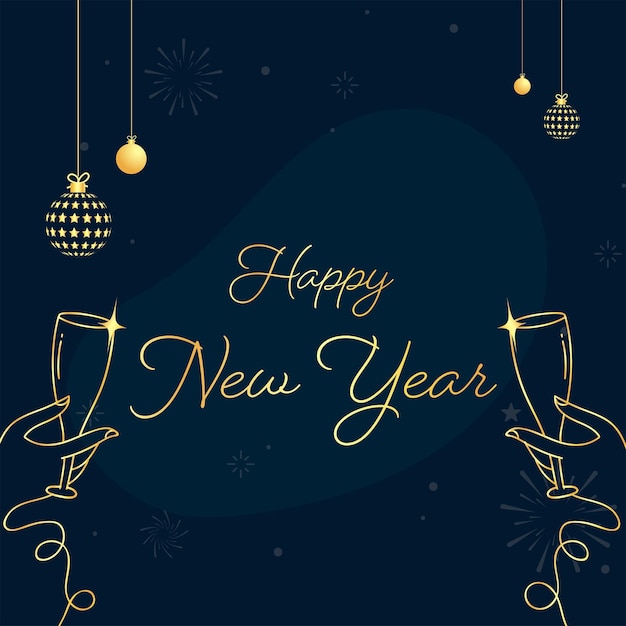The image features a dark navy blue background adorned with subtle bursts of star-like fireworks. At the center, "Happy New Year" is elegantly written in gold cursive script. Surrounding this festive message, two hands outlined in gold hold champagne glasses from either side at the bottom. Additionally, the top of the image showcases thin gold strings suspending a series of Christmas ornaments. To the top left, there are two ornaments: one with a dark blue background decorated with gold star stripes, and the other, a small, simple gold bulb. A similar arrangement can be seen on the top right, with both ornaments appearing smaller. Overall, this detailed graphic illustration could serve as a holiday decoration, a cocktail napkin, a piece of wall art, or even an e-card, exuding a warm, celebratory feel with its neon-like design elements.